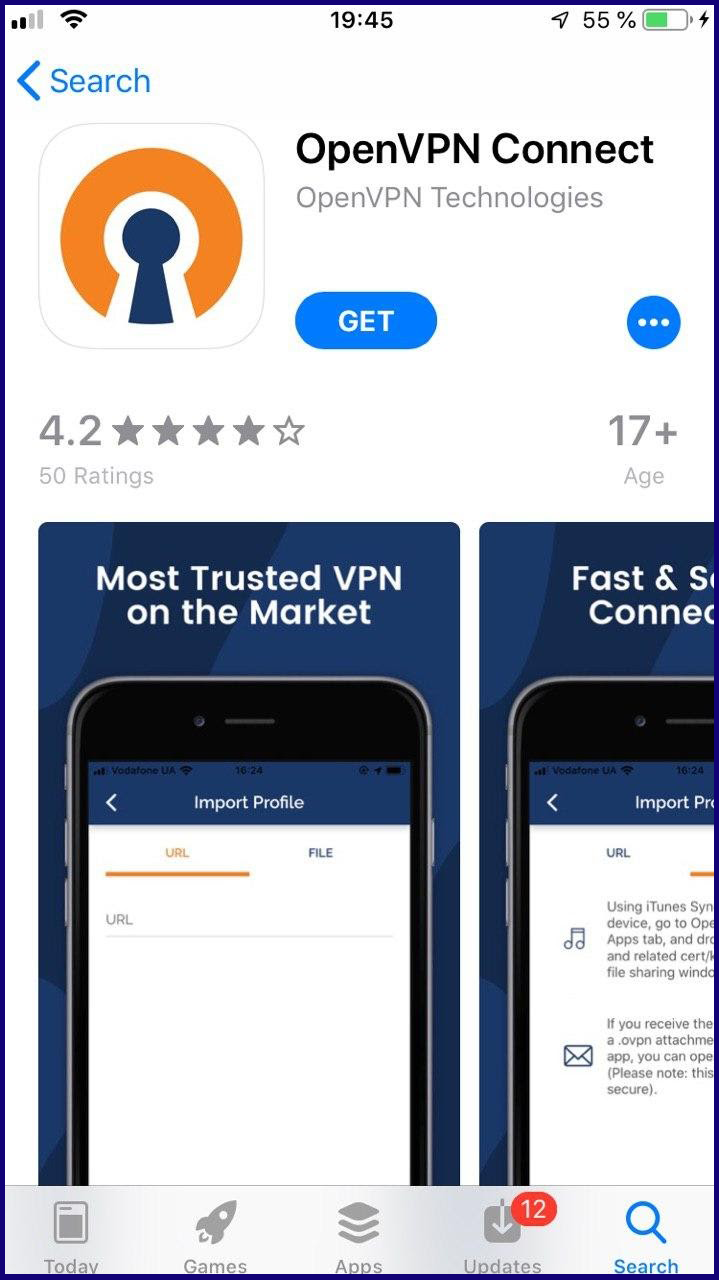This image is a screenshot captured from a smartphone, which features a predominantly white background. At the top of the screen, the battery icon indicates a 55% charge level, and the time displayed is 19:45. Below the time, the header signifies that this image likely originates from the Google Play Store if it's an Android device, or the Apple Store if it’s an iPhone. 

Central to the image is the application 'OpenVPN Connect'. To the left of the app name, the OpenVPN Connect logo is displayed prominently. The logo consists of a golden circle encircling a keyhole symbol. 

Underneath this, the screenshot displays part of the app's interface. The primary background within this section is navy blue with white text boldly claiming "Most Trusted VPN on the Market." Adjacent to this on the right is another partially-visible screenshot with a blue background, which extends beyond the right edge of the image, cutting off some of the view.

The image effectively showcases the main promotional and interface elements of the OpenVPN Connect app within an app store environment.